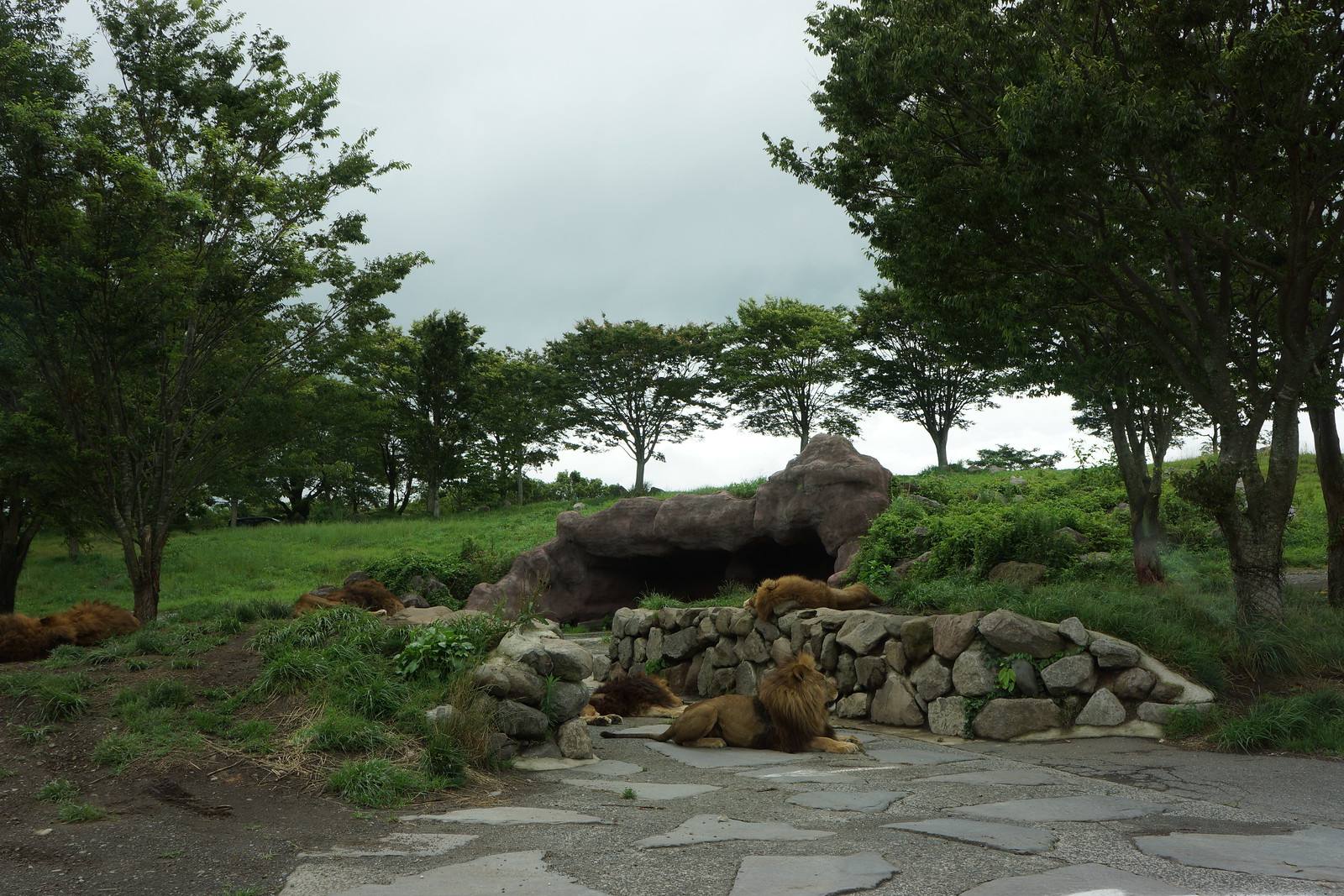This photograph depicts a serene scene within what appears to be a wildlife refuge or park. Dominating the foreground, a male lion with a stately mane lies comfortably on a rustic paved area composed of flat, artificial pavers. His paws are outstretched, and he is basking in the sun. Behind him stretches a rock wall made of boulders, providing a naturalistic backdrop. Atop this rock wall, another lion, possibly a female, can be seen resting. In the background, the landscape transitions to a picturesque hillside adorned with lush greenery and semi-circular arrays of fairly young trees. The sky is a clear blue, further enhancing the natural beauty of the scene. Additionally, there is a small rocky area that resembles a cave, offering potential shade and shelter for the animals. This idyllic setting, combining elements of both man-made and natural features, captures the essence of a tranquil wildlife sanctuary.